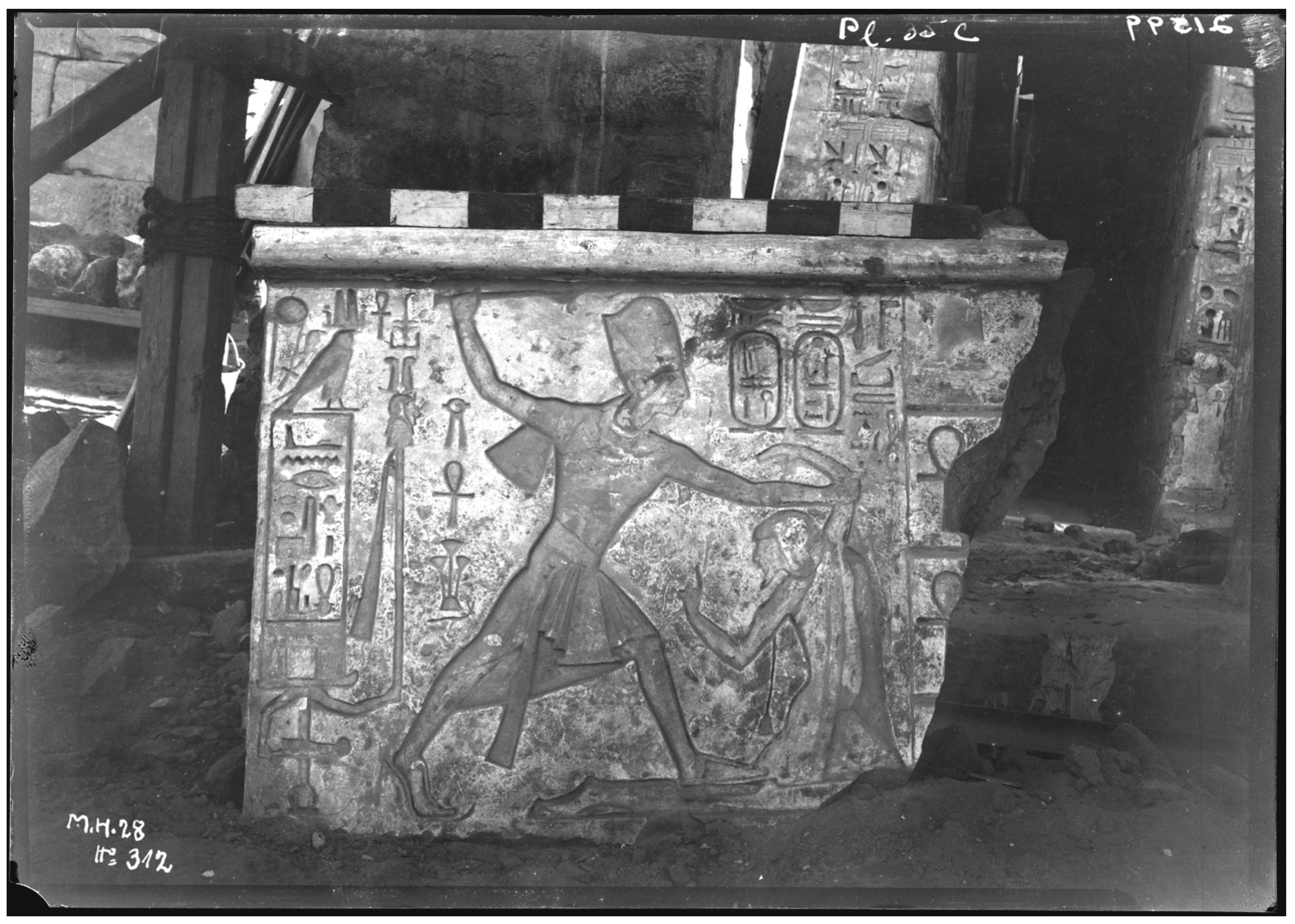This black-and-white photograph captures a broken and jagged slab of stone, likely an ancient Egyptian artifact or portion of a building. The weathered stone, covered with hieroglyphics and various symbols, depicts a dramatic scene where a pharaoh, standing aggressively, confronts a kneeling figure in a surrendering position, suggesting a scenario of punishment. In the center, the pharaoh holds tools or weapons, while an ankh and other runic symbols dot the surrounding hieroglyphics. The background of the image, resembling an excavation site, features rocky ground and what appears to be scaffolding and totem-like structures made of rock or concrete, supported by wooden posts and bearings. Notably, the bottom left corner of the photograph bears the inscription "MH 28 312" alongside an obscure symbol, with additional barely discernible numbers and letters at the top right, hinting at cataloging for museum or archival purposes.